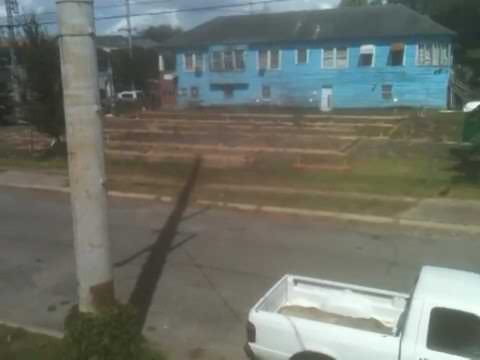The photograph, likely a screenshot from a video or security footage, depicts a suburban scene with a somewhat blurry quality. Dominating the background is a large, wide, two-story blue building with numerous windows, suggesting it might be an apartment complex or a duplex. The building features a grey to black rooftop. In front of the building, there's a mix of bare ground and patches of grass or farmland, with some unclear tan areas. The middle ground of the image presents a grey asphalt road, with the shadow of a light or telephone pole stretching across it from the left side. In the bottom right corner, a white pickup truck is partially visible, showing part of its cabin and the empty truck bed. Additionally, there's a glimpse of a white car parked near the building. The distant background includes a bit of blue sky and some electric lines, while the overall cloudy weather and the shadows indicate it's probably midday.